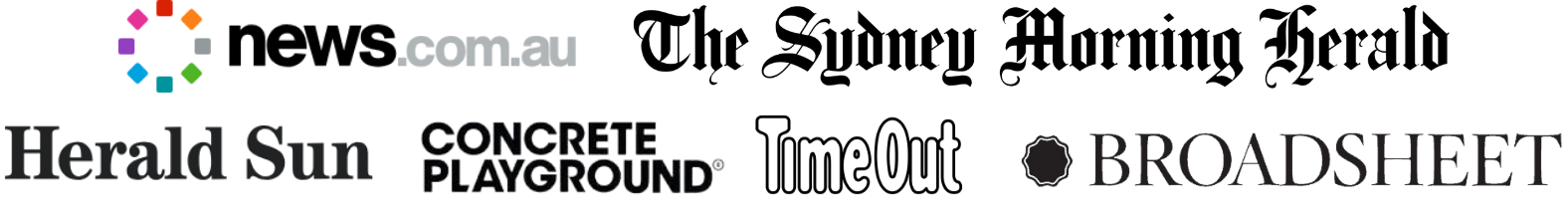The image features a white background adorned with numerous newspaper headers, each representing various media organizations in Australia. Among these, "Onews.com" stands out with its unique logo—a series of colors forming an 'O' followed by the word "news.com." Another prominent header is the "Sydney Morning Herald," presented in an old-fashioned, bold black font, reminiscent of the typography used by the Detroit Tigers. 

The next line showcases four different media organizations, starting with "The Herald Sun," which is displayed in a thick, bold black font. Following this is "Concrete Playground," featuring its name with the word "Concrete" positioned above "Playground," and includes a registered trademark symbol. Next is "Time Out," characterized by its white, or perhaps open, lettering outlined in black. Finally, the header for "Broadsheet" grabs attention with an all-caps, black and white design, accompanied by a logo resembling a blossom located to the right of the text.